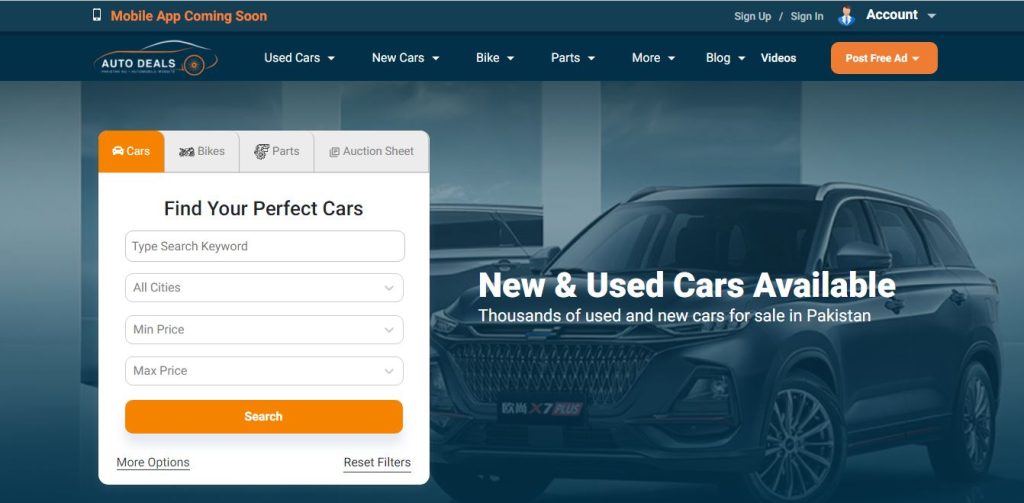This horizontal image, likely viewed from a computer or smartphone, captures a webpage featuring a comprehensive online automotive marketplace with a sleek, dark gray rectangular strip at the top. In the upper left corner of the strip, there is a phone icon accompanied by an orange message announcing, "Mobile app coming soon." On the far right, there's a "Sign up/Sign in" link with a person icon, an "Account" dropdown menu indicated by a white arrow pointing downward.

Beneath this header is a near-black rectangular navigation bar. On the left side of this bar, a car icon labeled "Auto Deals" is displayed. Running across the bar are clickable white options: "Used Cars," "New Cars," "Bike," "Parts," "More," "Blog," and "Videos." Adjacent to "Videos" is an eye-catching orange button that reads "Post Free Ad" in white letters.

The main content area features a white box over a background image of cars in grayscale. Overlaying the background is bold text stating, "New and Used Cars Available," with a subheading, "Thousands of used and new cars for sale in Pakistan," in slightly lighter font.

Within the white box, the highlighted option "Cars" is displayed in orange, with other options for "Bikes," "Parts," and "Auctions" available for selection. Below this, the text prompts "Find your perfect cars," and a search interface follows, allowing users to enter search keywords, select from "All cities," and input minimum and maximum price values. A prominent orange "Search" button facilitates the search process. Additionally, underneath this search section, users can access "More options" on the left or "Reset filters" on the right, both underlined for emphasis.